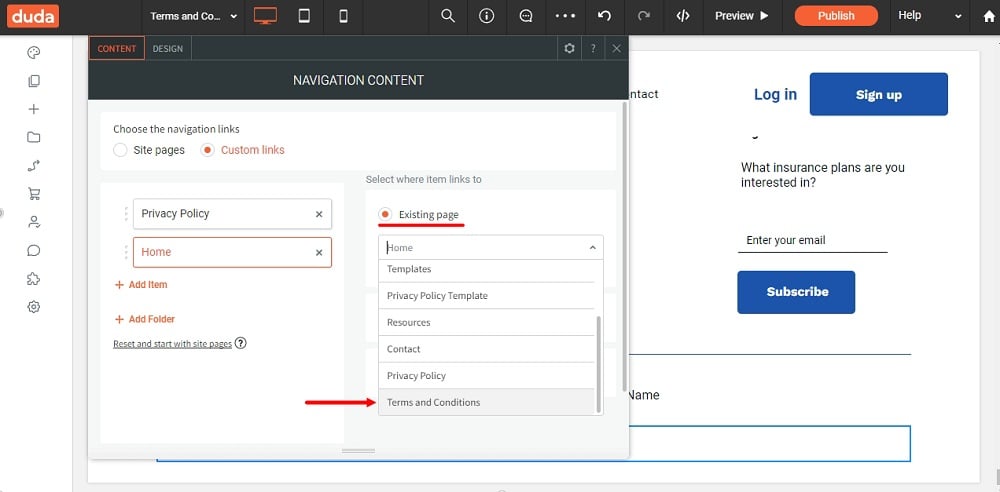The image showcases a webpage with a sophisticated layout, predominantly framed by various colored borders and text. At the very top, a black border spans the width of the page, housing an orange rectangle in the left corner with the bold, white text "DUDA". To the right of this logo, white text reads "Terms and Co...".

Immediately below the top border, several icons and tabs are lined up: an orange laptop monitor, a white-outlined cell phone monitor, a white-outlined battery icon, followed by approximately eight additional tabs. Further across, a refresh button and a search icon are present. A white "Preview" tab is adjacent to an orange "Publish" tab with white text. Further right, the "Help" option appears before reaching the home icon, located at the extreme right corner.

On the left side of the page, under the "Data" section, there are nine clickable icons. Moving to the right from these icons, there is a thin gray vertical border, followed by a black border. In the left corner of this black border, the word "Content" is highlighted in orange, while "Design" is displayed in black text. Centrally, the section features the white text "Navigation Content" with various related options underneath: Homes, Existing Pages, Choose Navigation Links, Custom Links, and Site Pages. 

Another thin gray border transitions to a white background area. In the middle of this section, a blue text field is labeled "Login". Below it, a blue tab with white text says "Sign Up". Small black lettering beneath this asks, "What insurance plans are you interested in?" Above a designated input line for email entry, there are black instructions noting, "Enter your email." Finally, a blue "Subscribe" button with white text appears, and at the bottom left corner of the page, the word "Name" is displayed.